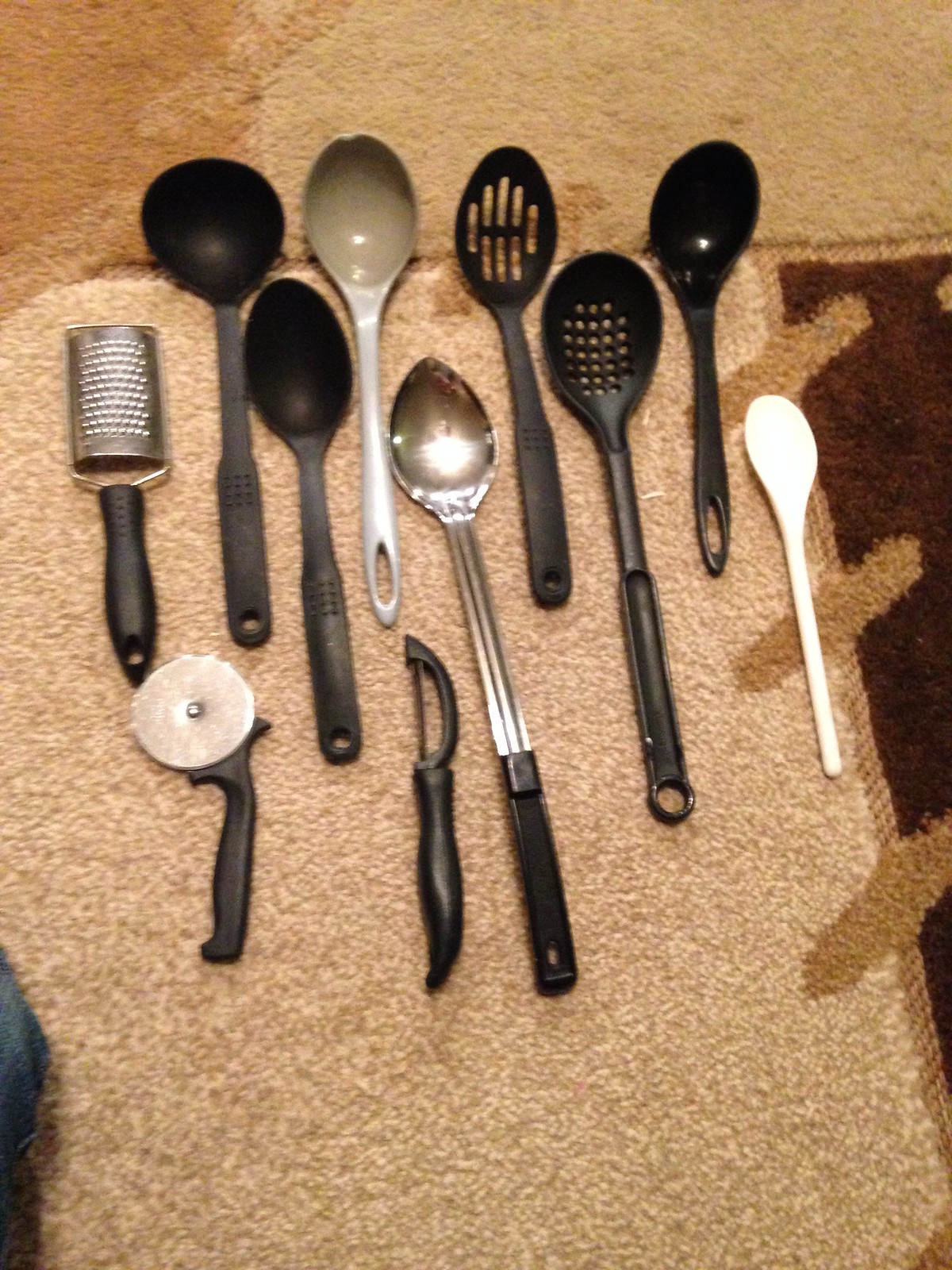The photograph showcases an array of various kitchen utensils placed on a carpeted floor. The carpet features a tan color with a slightly darker brown diagonal pattern, transitioning into a deeper brown section on the right. Scattered across the carpet are different kitchen gadgets and accessories, including several black plastic spoons and ladles. Among them are two black slotted spoons, one with hollowed-out circles, and a black ladle for soup. There is also a large silver ladle with a black handle, a black vegetable peeler situated at the bottom of the frame, and a white plastic spoon with a wooden-like handle and a rubberized end. On the left side of the image, a black-handled cheese grater and a black-handled pizza cutter are visible. The items are arranged in a somewhat organized manner, although not in a strictly straight line.